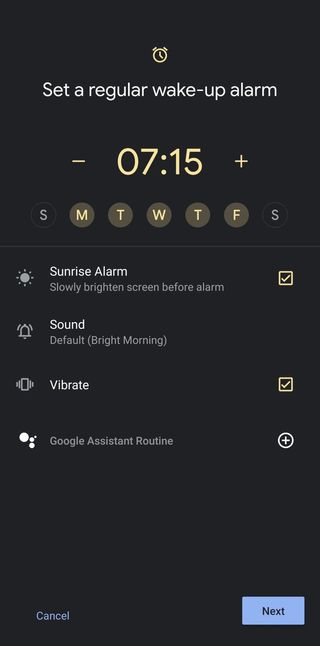The image captures a mobile phone alarm setup screen against a black background. At the top, a clock icon is centrally positioned, followed by centered white text stating, "Set a regular wake-up alarm." Below, a large yellow time display reads "07:15," flanked by a minus sign on the left and a plus sign on the right to adjust the time. Further down, there are seven circular bubbles each indicating a day of the week, labeled S, M, T, W, T, F, S. The bubbles for Monday (M), Tuesday (T), Wednesday (W), Thursday (T), and Friday (F) are highlighted in brown, indicating the alarm is set for these days. 

Directly below these weekday indicators, on the left side, are three options with accompanying icons and checkboxes: 
1. "Sunrise alarm," with the description "slowly brighten screen before alarm," is checked.
2. "Sound," set to the default option.
3. "Vibrate," which is turned on.

At the bottom left of the screen, there are two buttons: one labeled "Cancel" and the other on the bottom right labeled "Next."